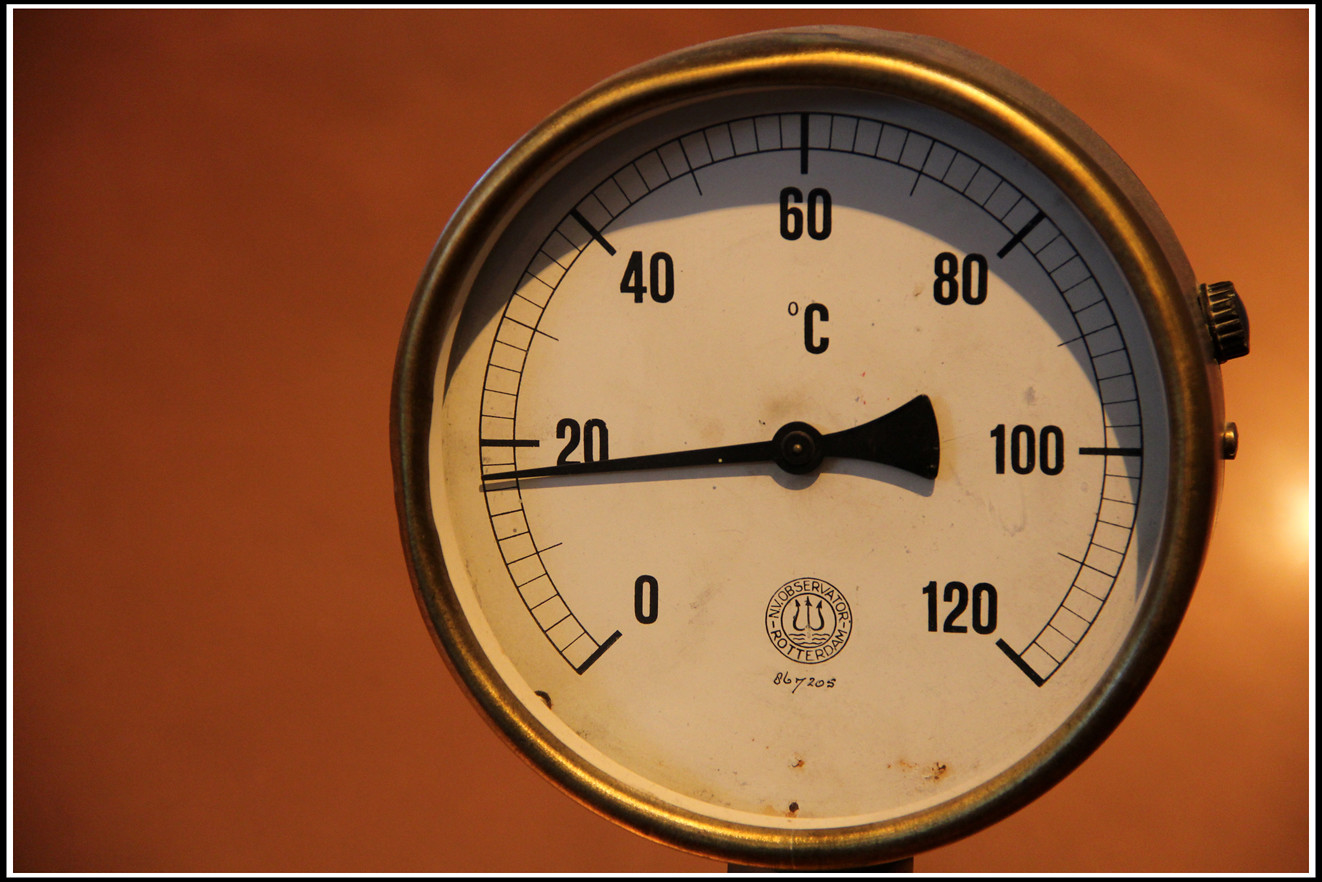The image is set against a background featuring a unique shade of brownish-red, transitioning into a shadowed area in the upper left corner. On the right side, a small circle of light brightens the scene slightly. The focal point of the image is an old-fashioned device resembling a clock but actually serving as a thermometer. 

This thermometer features a small circle next to a bold letter 'C'. The temperature scale begins at zero and increments in intervals of 20: 20, 40, 60 at the top center, 80, 100, and finally 120. Unlike a typical clock, these numbers represent temperature measurements rather than hours. The long black hand of the thermometer points just below the number 20.

Beneath the black hand, there is an emblem depicting a circle with a pitchfork-like symbol inside it. Below this emblem, some cursive writing can be seen, adding further character to this vintage device.